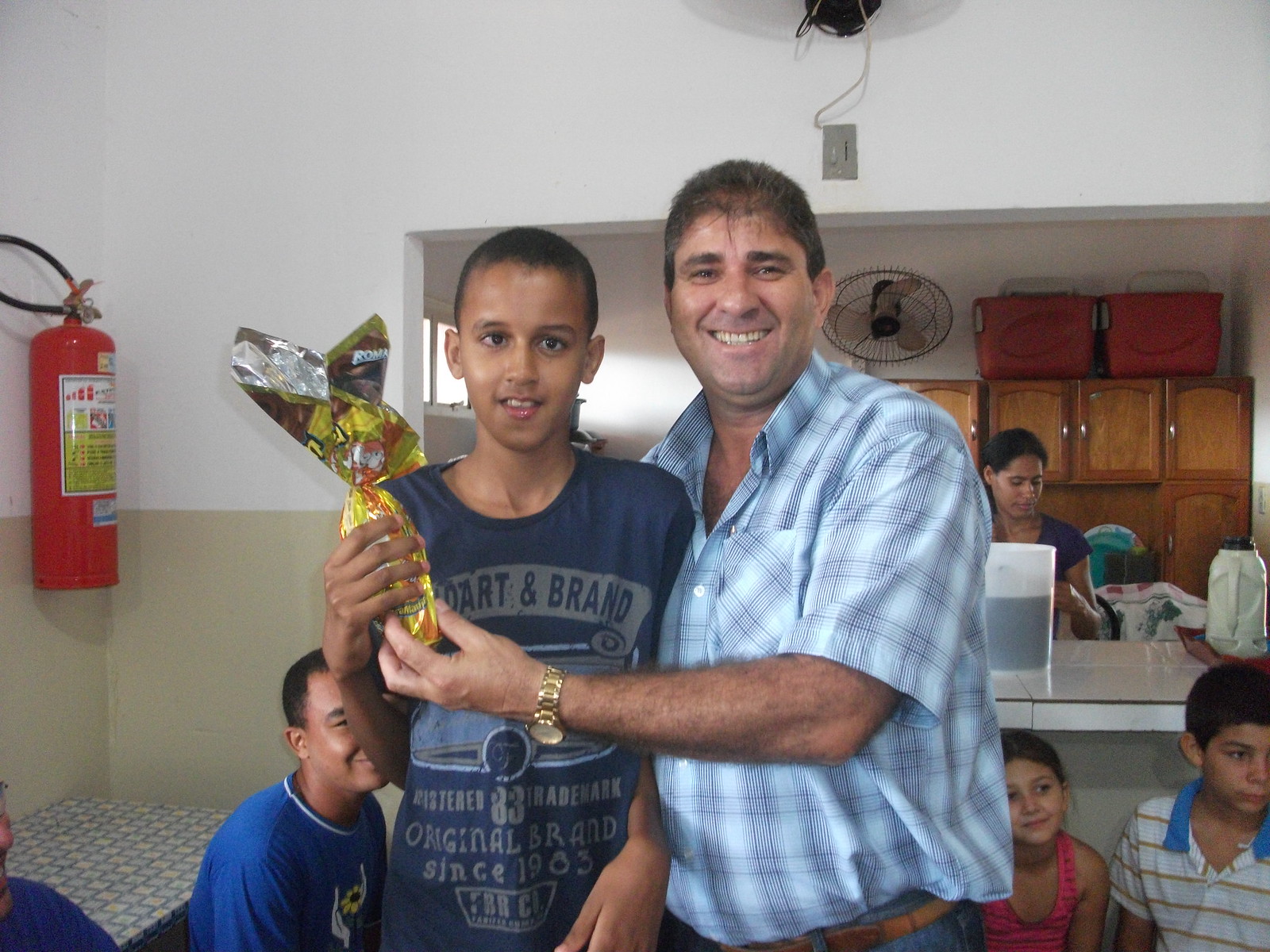In this image, we see a cheerful scene inside a home, likely a kitchen or living room, with white walls and brown cabinets. At the forefront, a young boy with short black hair and brown skin is wearing a navy blue t-shirt. He stands next to an older man with thinning, greying hair, who is wearing a light blue checked shirt, blue jeans, and a brown belt. Both individuals are smiling broadly and are jointly holding a shiny, gold foil-wrapped object, which appears to be a bottle or an award.

In the background, there's a gathering of people, adding to the lively atmosphere. Among them are two children and three adults seated, all smiling. Notably, a young girl in a pink top and a boy in a polo shirt can be seen. Further back, near the kitchen area, a woman is engaged in some activity near the countertop. This kitchen area is equipped with dark brown cabinets and a white, shiny countertop. Mounted on the wall to the left is a fire extinguisher, and atop the cabinets are a large round fan and two sizeable red coolers. The scene exudes a sense of celebration and community as everyone seems to be enjoying the moment, posing for the photo.